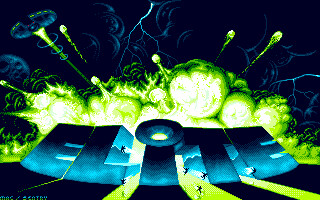The image appears to be a digital artwork characterized by a predominantly dark background, which sets a dramatic tone. The centerpiece of the image features vibrant, green, neon-like, nuclear bubbles that seem to radiate an intense, almost explosive energy, illuminating the scene from behind. In the foreground, the word "ELITE" is prominently displayed in bold, block letters, rendered in a deep blue with darker shades adding depth. The letters are stylized with a slight curve, giving them a dynamic, almost three-dimensional effect. Green light from the background seeps through the open spaces within the letters, enhancing the ethereal glow. Additionally, green fireballs shoot out from various points, reflecting the mysterious and powerful energy emanating from the background. The overall composition suggests a sense of grandeur and intensity, making the visual both intriguing and captivating.